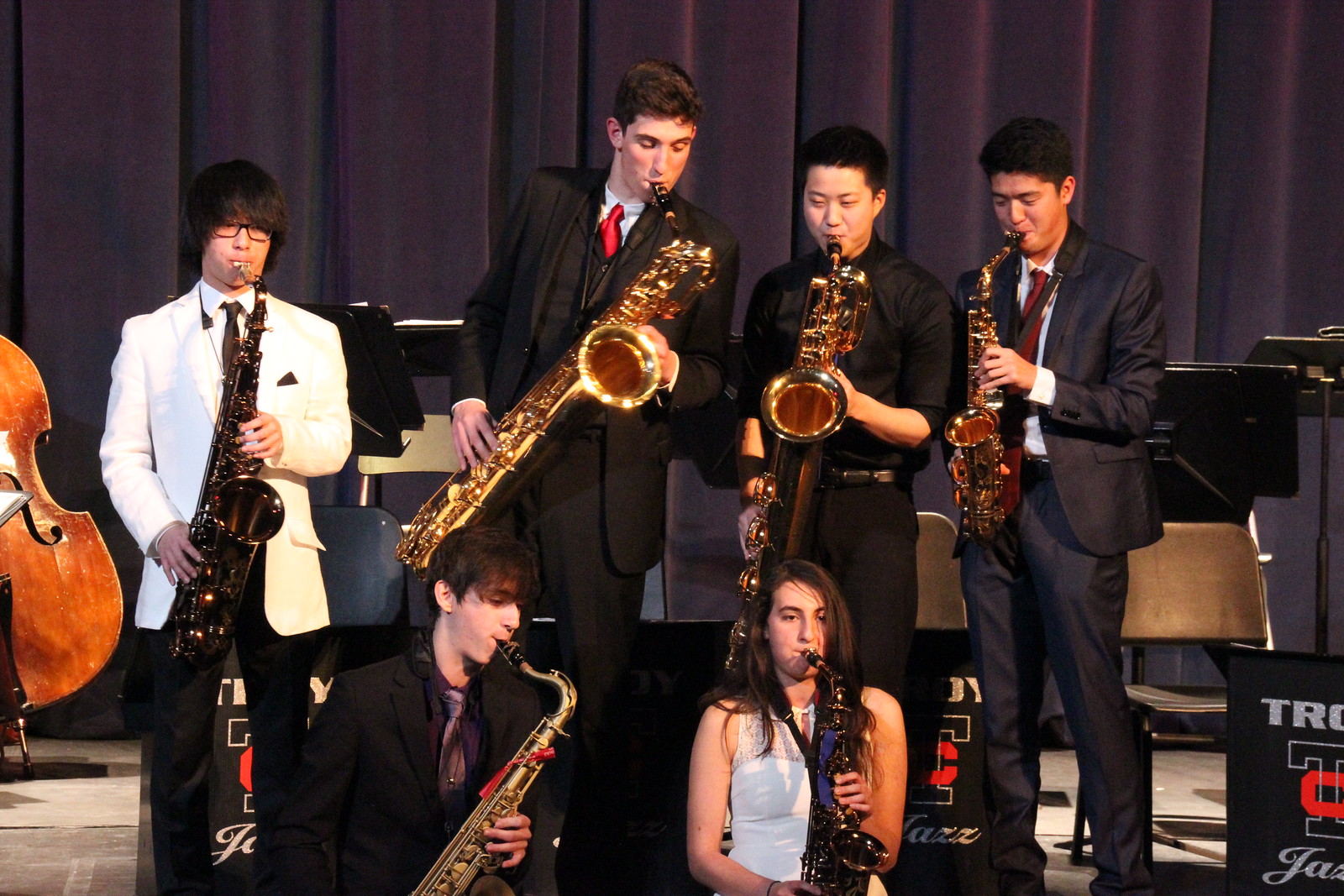This image captures a jazz ensemble from Troy University performing on stage. The floor is a light, off-white color, and the backdrop features a tall, black stage curtain. The ensemble consists of six saxophonists: five men and one woman. In the forefront, standing from left to right, are four male musicians. The first is dressed in a white suit coat with black pants and a dark tie, followed by three men in black suits; two of them are wearing red ties, while the tie of the third is obscured by his saxophone. In the lower center, a man in a black suit with a gray tie plays standing next to a woman in a white sleeveless dress. Visible off to the left is part of a double bass, though the bassist is not in the frame. Behind the musicians, chairs, music stands, and a black sign with partially obscured text are noticeable. The ensemble forms part of the Troy University Jazz band, as indicated by the writing seen in the image.